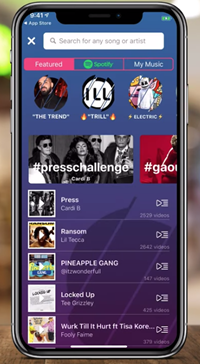Set against a vibrant and multicolored background ranging from ivory to dark gray and light gray, with a splash of neon green in the upper left corner, the image features a sleek silver cell phone standing upright in a vertical orientation. The cell phone screen is illuminated, displaying various app elements.

On the left side of the phone, there are three visible buttons, while the right side features a single button. Dominating the screen display is a blue background. In the upper left corner of the screen, the time is prominently shown as 9:41. Directly below the time, the words "App Store" are displayed, followed by a prominent white search bar filed with the text "Search for any song or artist."

Beneath the search bar, several options are available: "Featured," which is highlighted, a pink box labeled "Pink Box," and "My Music" to the right. Centered below these options is the "Spotify" logo.

Under the highlighted "Featured" section, it reads "The Trend," followed by "Tell," "Electric," and an image of a band. Below this, the text "Hashtag Press Challenge" is displayed, and beneath this headline lie five album covers with accompanying options to play the tracks displayed.